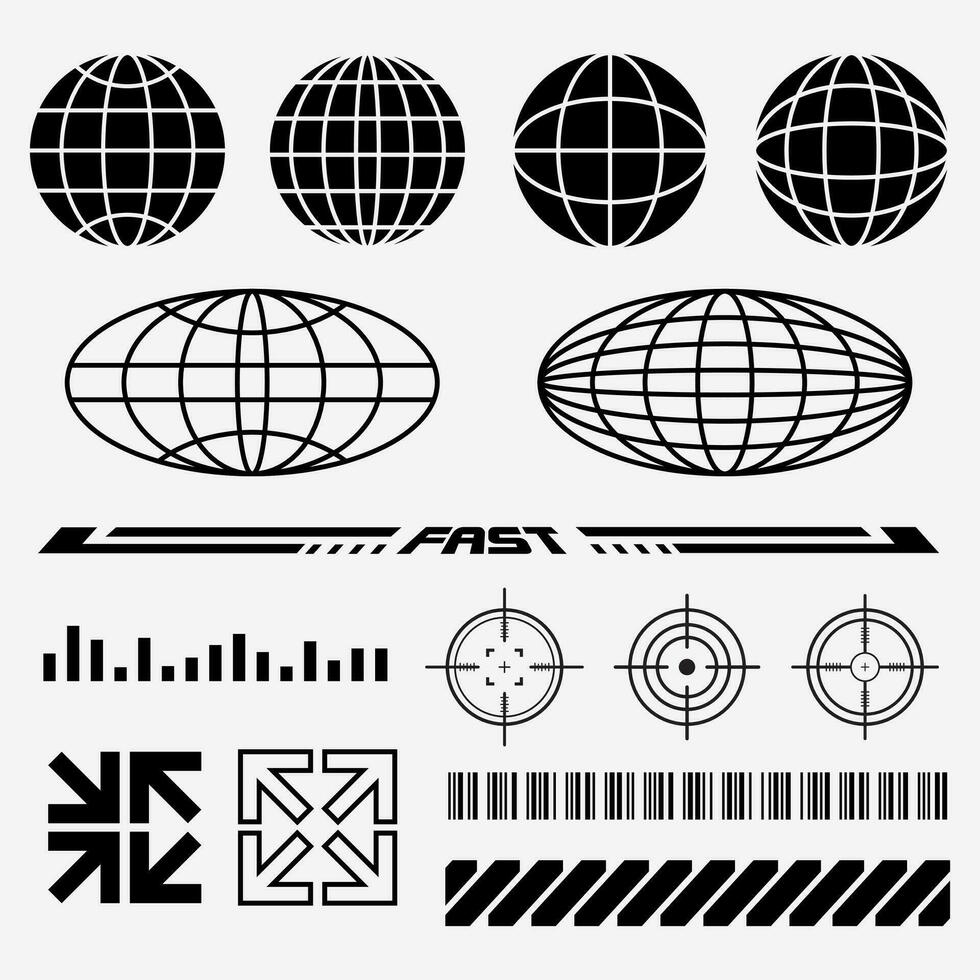Against a light gray background, there's an array of various black symbols. On the top row, there are four globe-like shapes, each with distinctive curved and horizontal lines reminiscent of geographic latitudes and longitudes. Below these, two elongated oval shapes feature different line patterns: the first has a combination of straight and curved lines resembling meridians, and the second is adorned with round lines that lend it a watermelon-like appearance. 

Further down, there's a bold black strip with the word "FAST" prominently centered. To the left of this, a cluster of vertical lines stands tall, evoking a bar graph. Adjacent to this, several circular symbols suggest bullseyes, each marked by lines pointing in four cardinal directions with a central spot. 

In the bottom left corner, a group of arrows forms a square, with their tips pointing in various directions. Next to this, another set of arrows, similarly arranged in a square, also points in different directions. Following this, a sequence of vertical black lines mimics the appearance of a barcode or QR code. Lastly, a set of black lines, slightly angled and leaning leftward, completes the composition.